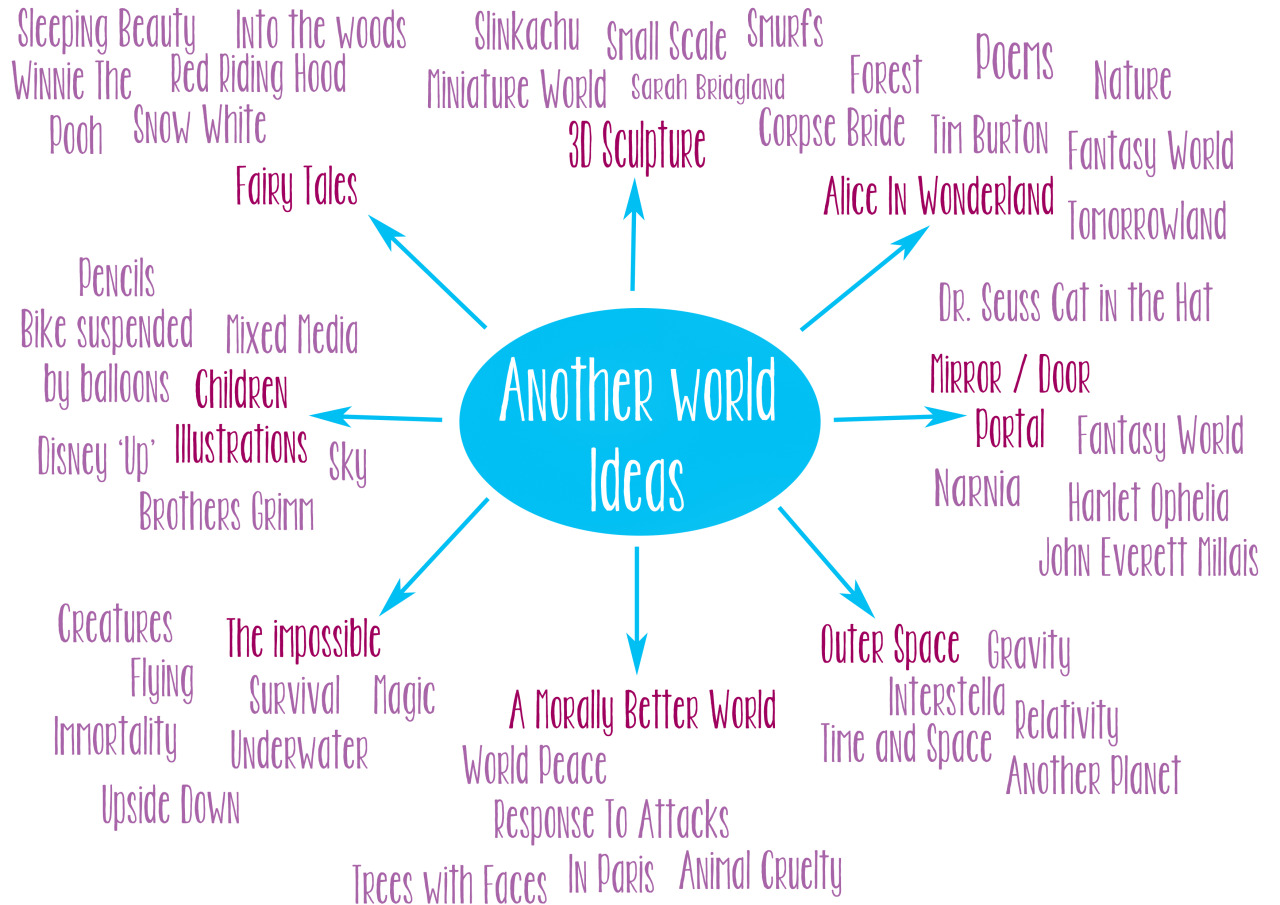In this image with a white background, the central feature is a blue oval containing the white text "Another World Ideas" arranged on two lines with "Another World" on the top line and "Ideas" on the second line. Radiating from this oval are eight arrows leading to various categories and associated terms. The top three arrows point to the upper left corner, directly upwards, and the upper right corner. Two arrows extend from either side of the oval. The bottom three arrows diverge towards the lower left corner, directly downward, and the lower right corner.

The categories and their detailed elements are as follows:
- **Fairy Tales**: includes "Sleeping Beauty," "Into the Woods," "Winnie the Pooh," "Red Riding Hood," and "Snow White." These terms are displayed in a dark burgundy color, while the connecting word cloud elements are in a lighter pink hue.
- **3D Sculpture**: features terms like "Slinkochu," "Small Scale," "Smurfs," "Miniature World," "Sarah," and "Bridgeland."
- **Alice in Wonderland**: associated with elements such as "Mirror," "Door," and "Portal."
- **Outer Space**
- **A Morally Better World**
- **The Impossible**
- **Children’s Illustrations**

Each category is represented by clusters of keywords branching from the primary blue oval, forming a comprehensive flow chart that visually organizes creative ideas derived from the concept of alternate worlds.